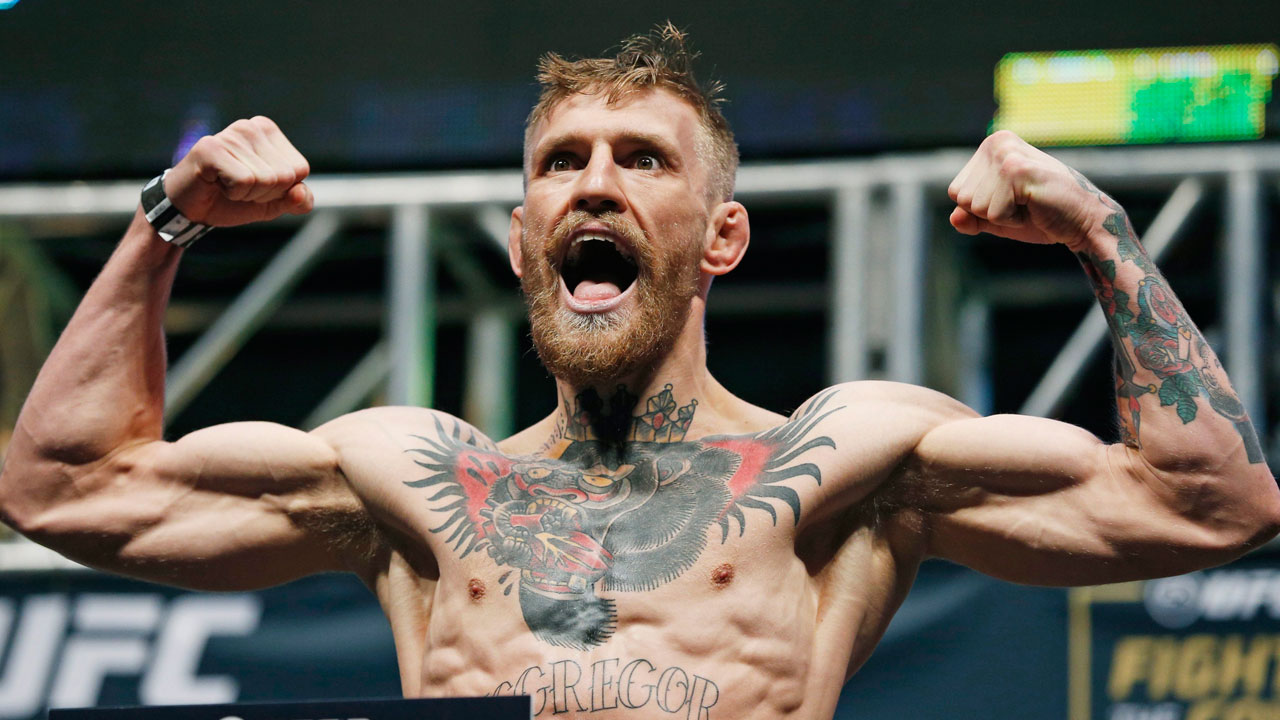This is a photograph of a mixed martial artist, likely UFC fighter Conor McGregor, prominently positioned in a stadium setting. The fighter has a tan complexion, with a red or brown beard and red hair, shaved at the sides. McGregor is captured with his arms raised, flexing his muscles, and his mouth wide open as if screaming or smiling at the camera. His right wrist sports a watch, and he has numerous distinctive tattoos. Across his neck and upper chest is a large tattoo of a bird with talons, predominantly black with red interior details, extending out to his shoulders. Below this, there is a black tattoo of his last name, "McGregor." Additionally, there is a tattoo visible on his left forearm. The background features a railing and banners; one to the left reads "UFC," and another to the right partially displays the word "fight" in yellow. Above McGregor, there is a green and yellow sign, adding vibrant color to the composition.